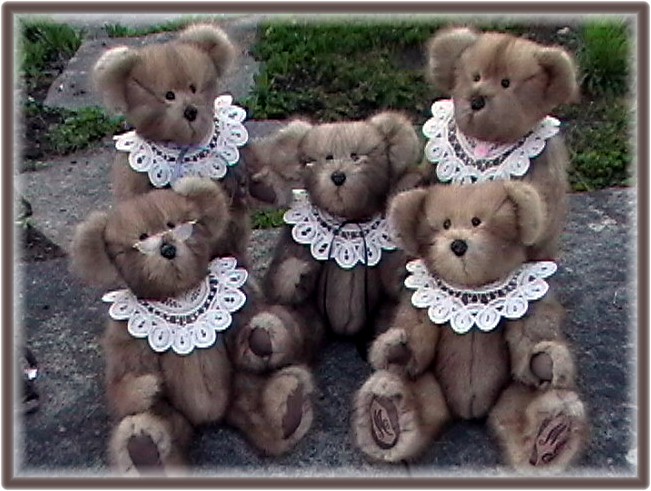In this outdoor color photograph, five posable teddy bears are arranged in a formation reminiscent of a family portrait. The bears, which all appear to be of the same model, are seated on a flagstone path, with a green lawn visible in the background. The bears have light brown mohair fur, black glass eyes, smooth light brown paw pads, and wear white lace collars. The central bear and the one in the lower left are adorned with wire-framed spectacles. Each bear has unique details: the top right bear has a pink rose appliqué on its collar, the top left bear sports a blue ribbon, and the middle bear has a trailing dark ribbon. The lower right bear features a monogram, which appears to be an 'N' or an 'M', on its paw pad.